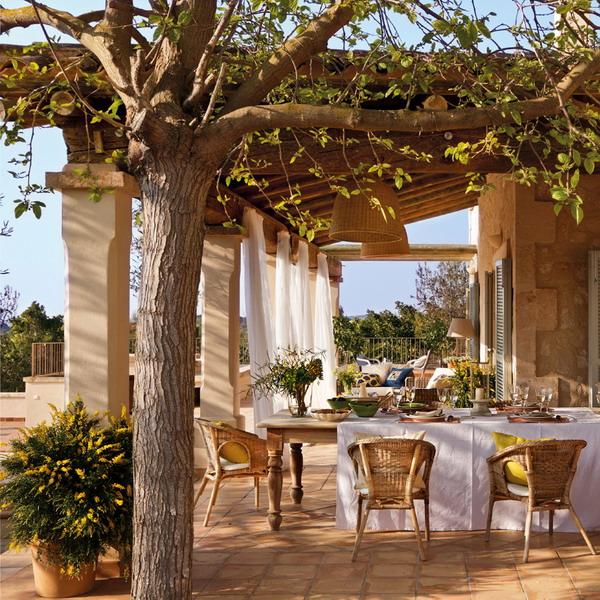This outdoor photograph captures an elegant and luxurious patio area, showcasing a beautifully designed setting under a rustic wooden pergola with white filigree curtains draped along tall vertical stone columns. The pergola, extending from a light stone house on the right, casts a charming and inviting atmosphere. 

Centrally, a long table adorned with an elegant white tablecloth features meticulous place settings, including beautiful plates, vases of flowers, and bowls, arranged in anticipation of a meal or event. The serene scene is enhanced by the absence of people, allowing the viewer to appreciate the preparatory grandeur of the occasion.

In the foreground, two chairs face the table while a third chair sits at the head, seen in profile. A tall tree with a canopy of green leaves and a light tan-colored clay pot with lush foliage further decorate the scene. Beyond the patio, a line of lush green trees outlines the horizon against a bright blue sunlit sky, with sunlight casting gentle shadows from the left onto the sand brown tiled floor of the patio, completing the picturesque setting.